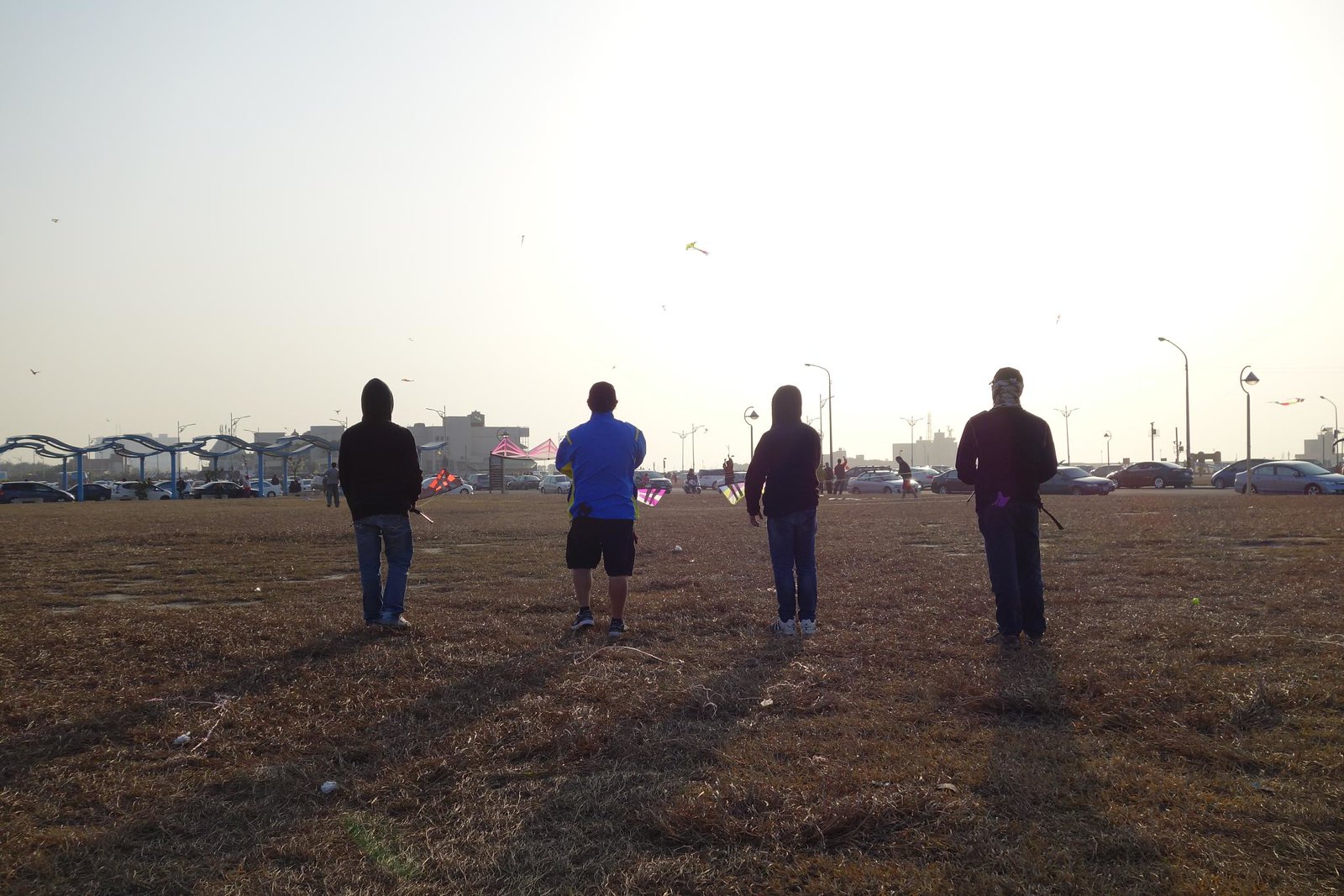In this color overexposed photograph, four young individuals stand in a large, grassy field, their backs to the photographer. They appear to be flying drones or radio-controlled airplanes, all gazing intently at the horizon. The group includes two people in hoodies, the first on the far left, who also wears blue jeans, and the third individual, who seems to be a child dressed in a dark long-sleeve shirt and blue jeans. The person second from the left sports a light blue t-shirt and black shorts, while the person on the far right, possibly a male, is clad in a long-sleeve maroon shirt and blue jeans. The setting includes a bright sky and a somewhat dark field. To the right, there are parked cars, streetlights, and a possible factory with a smokestack in the distance. On the left, additional cars are partially sheltered. Far in the background stands a structure with an undulating roof, likely a waiting area near a hotel or an airport.